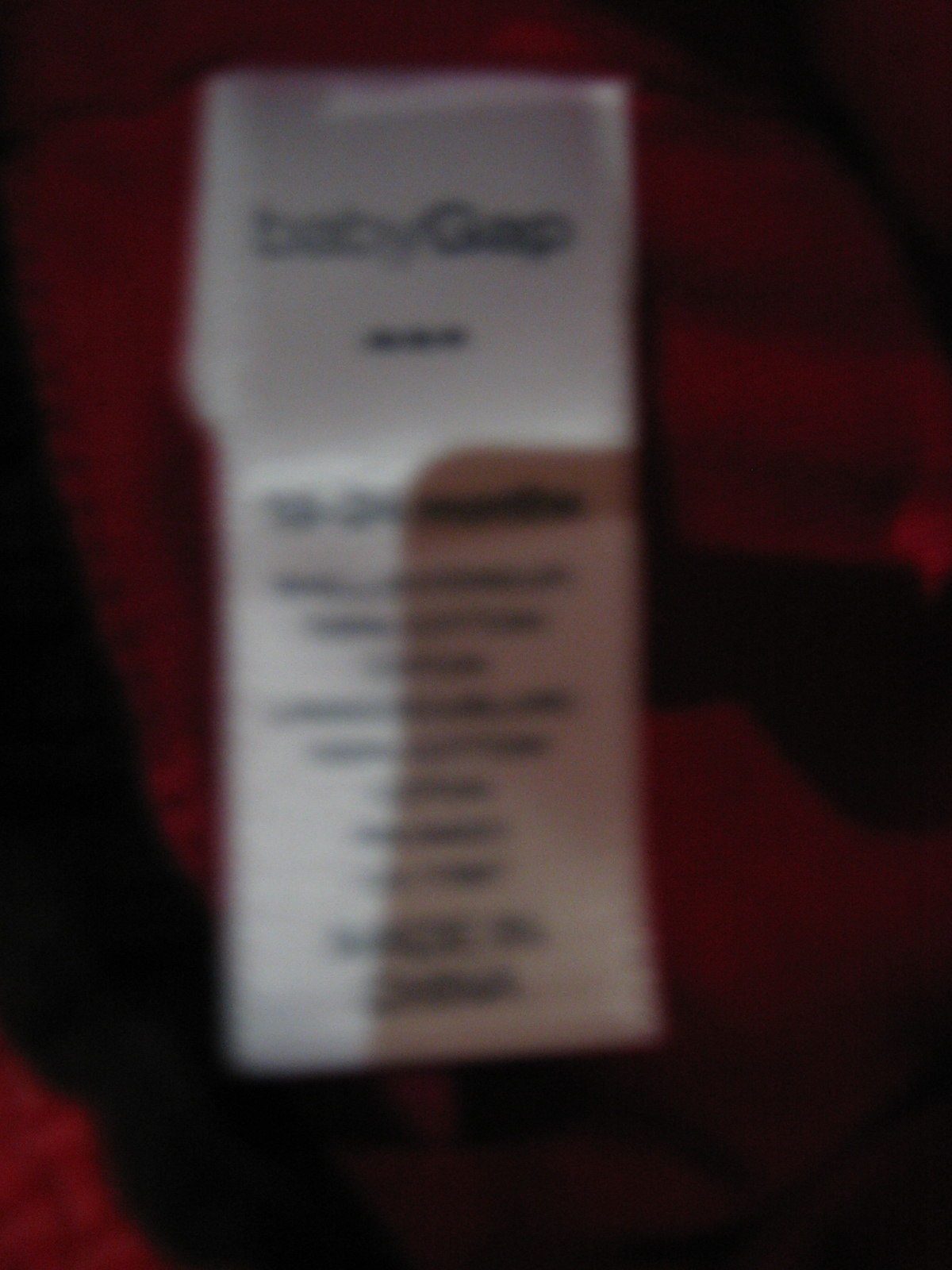An extremely blurry and out-of-focus image makes discerning details a challenge. Around the perimeter, patches of black, rusty brown, and brown hues come together in a chaotic blend. Dominating the center is a long, vertically-oriented rectangular shape, which appears to be a clothing label situated inside the neckline of a garment. Despite the severe blurriness, the most discernible element is the large black lettering at the top of the white tag, seemingly reading "Baby Gap". Below this text, the details are too small and blurred to decipher, though it likely contains fabric care instructions. The bottom right corner of the label is obscured by a shadowy, somewhat rectangular form, which masks part of the tag, further complicating the visibility.